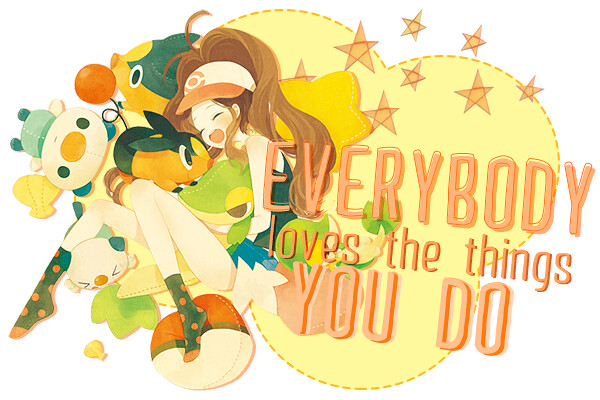In this softly colored illustration, a cartoonish girl reminiscent of Japanese anime style is depicted lying in a pile of varied stuffed animals. She has light brown, long hair flowing behind a white and orange cap, with a cheerful expression made more whimsical by her closed, smiling eyes. She wears a sleeveless green shirt, blue shorts, and calf-high green socks adorned with orange polka dots. The girl's slender legs and arms are curled up contentedly among the plush toys.

To her right, the background features a yellow cloud-like area composed of three intersecting circles, bordered by an orange dotted line. Above this, yellow stars are sketched in a playful, whimsical manner. Prominent orange text over this section declares, "Everybody loves the things you do." The entire illustration is rendered in soft, muted colors, adding to its overall charming and serene atmosphere.